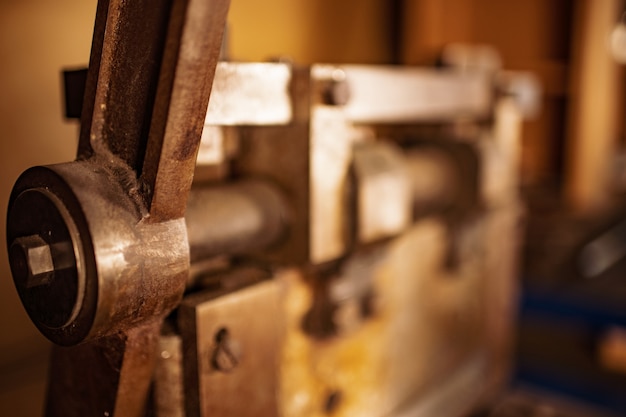The image features a highly detailed, close-up view of a metallic structure with the focused section occupying the left side of the frame. Dominating the foreground is a brown bronze-colored metal strut, featuring a central circular bracket into which another smaller circle is nested. This smaller circle is secured with a prominent metal nut, all appearing to be a seamlessly welded single piece. The strut itself extends diagonally across the image from the bottom left to the top right. 

The background is significantly out of focus, revealing a blurred industrial setting. There is a large cylindrical component and various interconnected metal objects. Some parts of the machine are visibly rusty, reinforcing its aged, heavy-duty, and industrial nature. Among the blurred details in the background, we can spot flat head screws, square and rectangular metallic elements, and an impression of orange walls. Additionally, faint blue lines and columns can be seen, along with some indistinct yellow instructions. The overall scene suggests an expansive and possibly antiquated machine, with parts exhibiting signs of prolonged use and wear.